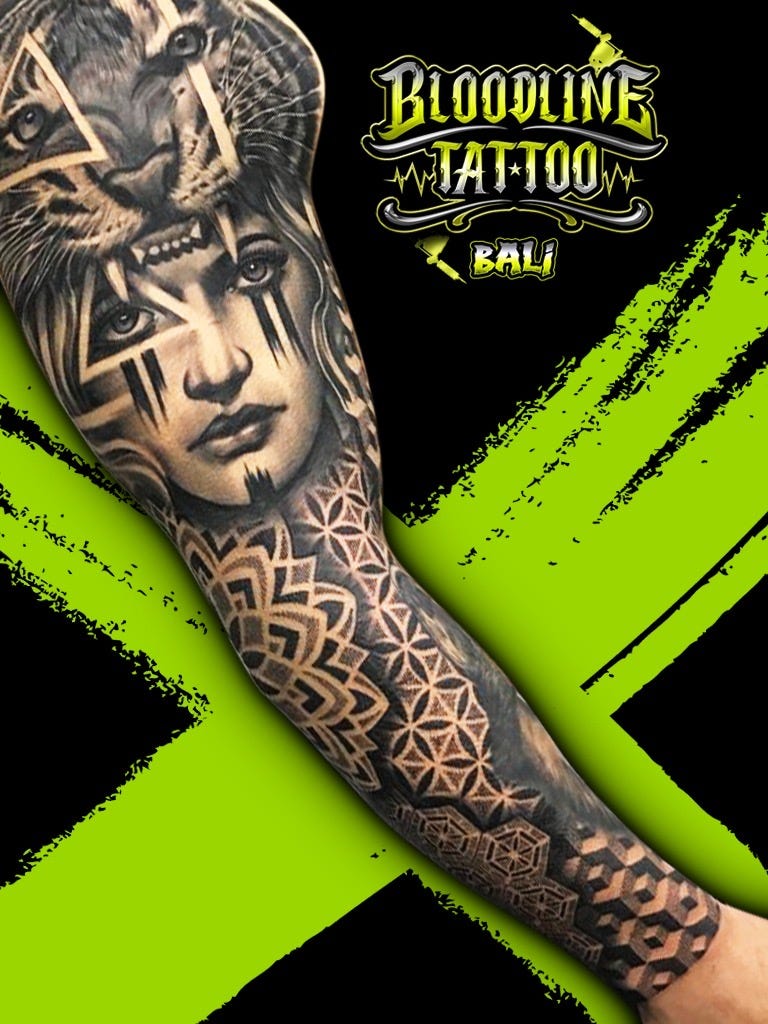The image features a black background with a prominent, bright green “X” accentuating the central tattooed arm. This arm, extending from wrist to shoulder, is adorned with an elaborate full sleeve tattoo. At the top of the shoulder is a striking black-and-white tiger, its mouth open and fangs bared, with a triangle by its left eye and a line through its right eye. Directly below the tiger, on the bicep area, is the detailed face of a woman, complete with red lipstick and lines extending down from her eyes. The forearm hosts an array of intricate designs, including a floral pattern on the elbow, honeycombs interspersed with flowers, and a cube pattern nearer to the wrist. In bright yellow lettering at the top right corner, the advertisement reads "Bloodline Tattoo Bali," with "bloodline" underlined and "tattoo" accompanied by an illustrative symbol resembling a tattoo gun. The vibrant green elements stand out sharply against the predominantly black background, drawing the viewer's focus to both the tattoo details and the branding.